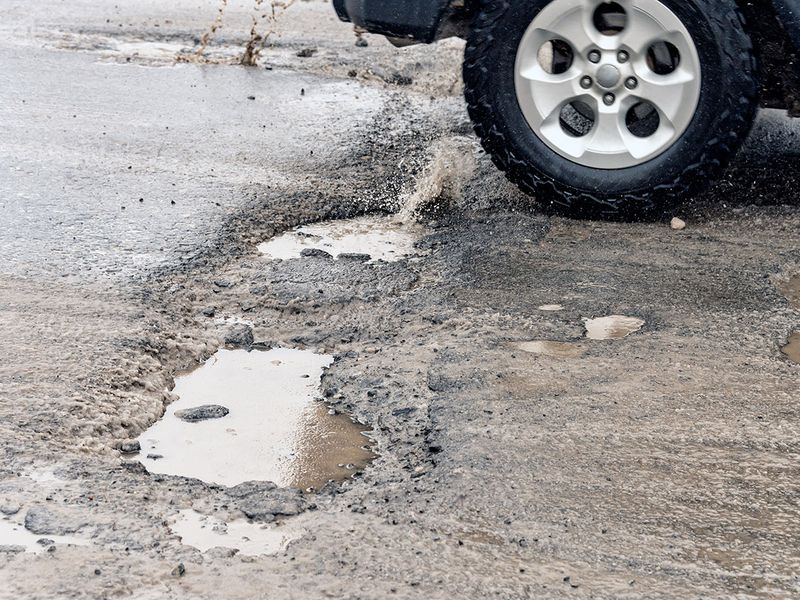In the image, we see a close-up of a deteriorating, muddy road, primarily focused on its worn and damaged pavement. The asphalt looks battered, with multiple potholes filled with muddy water, indicating heavy recent rainfall or a storm. The road’s surface is a mix of black asphalt and brown mud, scattered with stones and pebbles. One particularly visible pothole is brimming with stagnant water, further emphasizing the road's poor condition. A passing vehicle’s black tire with a silver rim is caught in action, splashing muddy water as it drives through one of the potholes, underscoring the impact of the rainfall. The scene is still under rainfall, evidenced by the small splashes in the puddles. This image vividly depicts the road's severe degradation and the challenging driving conditions it imposes.